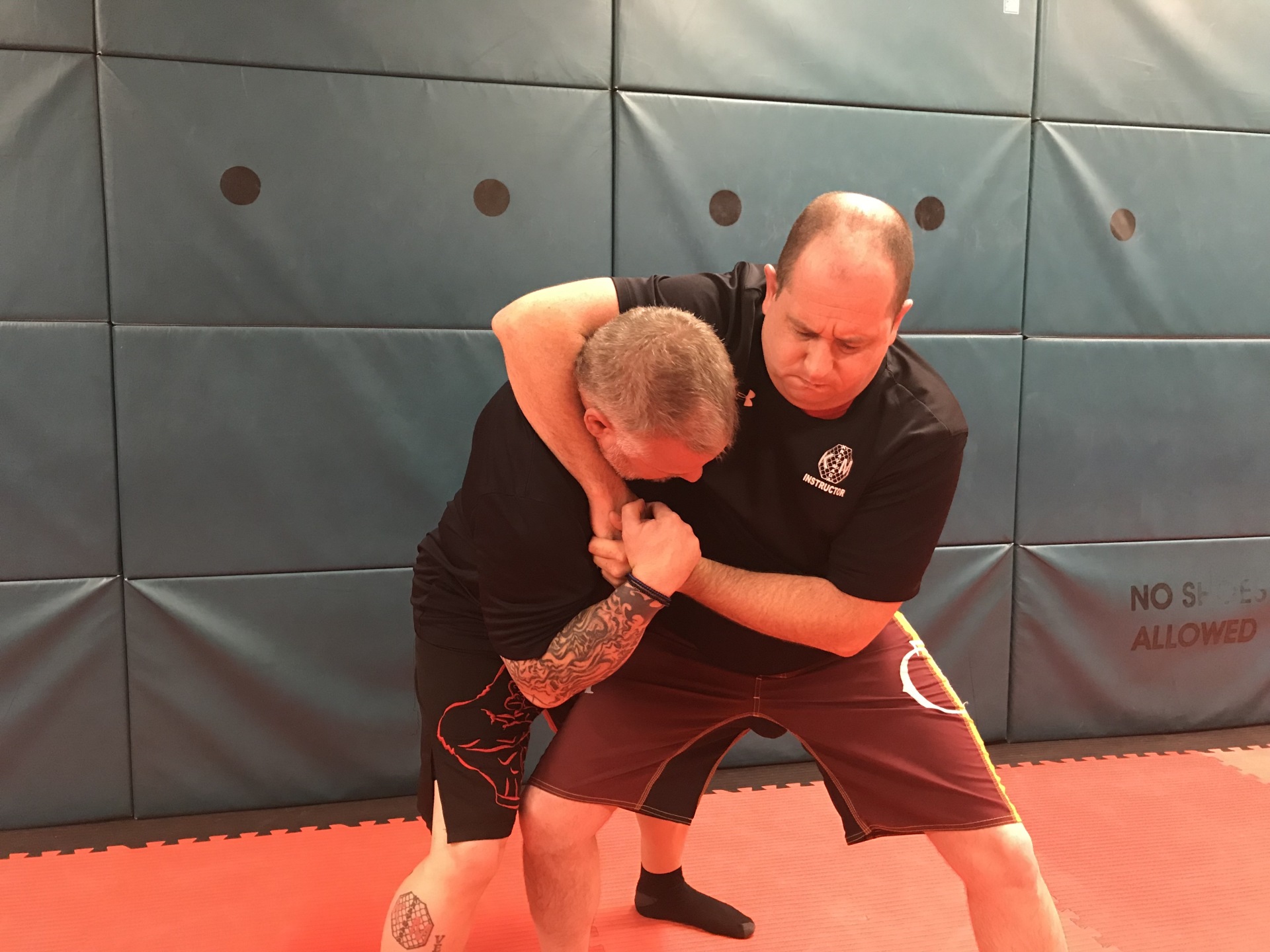In the image, we see two men wrestling inside a gym, where the primary focus is on the people rather than objects. Both men are positioned in the center of the photo, standing on a soft, orange mat that covers the bottom of the image. The man on the left, tattooed on his arm and leg, is dressed in a black t-shirt and red shorts with a white design. The man on the right, wearing a black t-shirt and black shorts with a red design, is holding the other man in a chokehold.

The background consists of dark bluish-green padded walls with rectangular sections, providing cushioning for the gym. Near the bottom right of the padding, there are a couple of black circles, and the text “no shoes allowed” is visible in the bottom left corner of the image. The colors in the scene include green, white, black, tan, gray, red, orange, maroon, and brown, with the floor’s padding extending from an orange hue to a brown border. This setting is clearly within a gym or a wrestling facility.